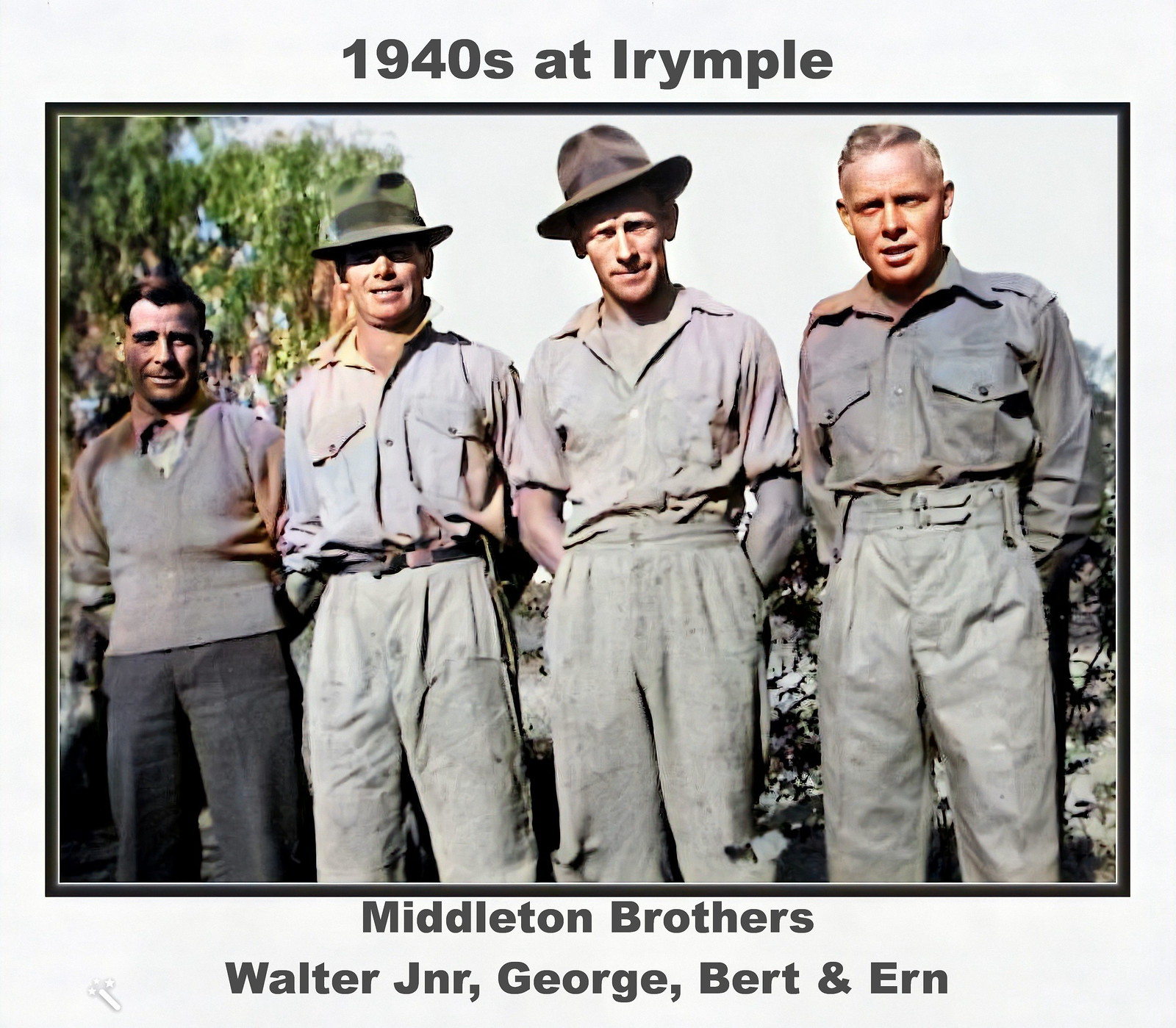This photograph, bordered in black with an off-white, slightly gray background, presents a retouched or enhanced image from the 1940s taken at Irymple. The photograph features four men, identified by the caption at the bottom as the Middleton Brothers: Walter Jr., George, Bert, and Ern. All four men stand in a line with their hands behind their backs, with two of them donning hats and two of them not. Their attire consists of what appears to be work clothes, except for the man on the far right, who is wearing a sweater. The outdoor setting includes visible bushes behind them and a glimpse of trees in the top left corner. The text above the photograph reads "1940s at Irymple," while the text below confirms their identities.